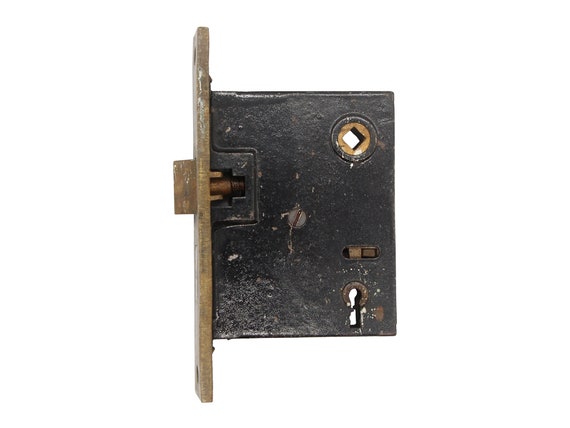This image depicts the side view of a door lock mechanism removed from the door. The lock is rectangular in shape and primarily metallic, with a side section showing a brown, slightly dirty wooden part. The mechanism consists of various components including a keyhole, a metal bolt, a lever, and another dial. The keyhole opening is visible on the metal surface, highlighting its key function. The image is set against a simple white background, emphasizing the intricate details of the lock’s inner workings that would typically be embedded within the edge of a door, where it interacts with the door jamb to secure the door when closed.